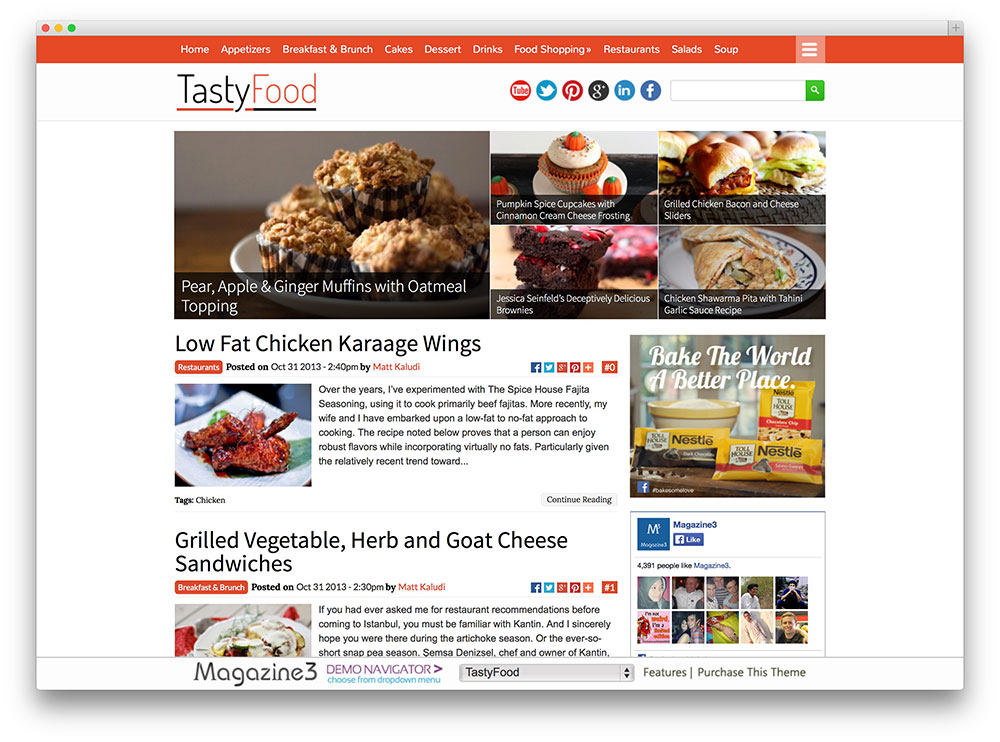The website appears to belong to "Tasty Foods" and features a clean, white background with a thin orange line at the top. Approximately five inches from the left, the logo prominently displays "Tasty Food" with "Tasty" in black text above an orange line and "Food" in orange text above a black line. 

On the right side of the header, social media icons are neatly arranged within circles: YouTube, Twitter, Pinterest, Google Plus, LinkedIn, and Facebook. Adjacent to these icons, a search bar features a green box with a magnifying glass icon.

The main body of the page displays various food images accompanied by descriptive text. The largest image shows muffins labeled "Pear, Apple, and Ginger Muffins with Oatmeal Toppings," with the text overlaid in white. Below this, four smaller images of equal size present diverse recipes: 

1. A single cupcake labeled "Pumpkin Spice Cupcakes with Cinnamon Cream Cheese Frosting."
2. "Grilled Chicken Bacon and Cheese Sliders."
3. "Jessica Seinfeld's Deceptively Delicious Brownies."
4. "Chicken Shawarma Pita with Tahini Garlic Sauce Recipe."

Additionally, an image showcases "Low-Fat Karachi Wings" accompanied by a brief excerpt from the author. An advertisement for Nestlé Toll House chocolate chips is also present. Most of the font on the page is in black, and several buttons categorize the content, presumably by restaurant or recipe type.